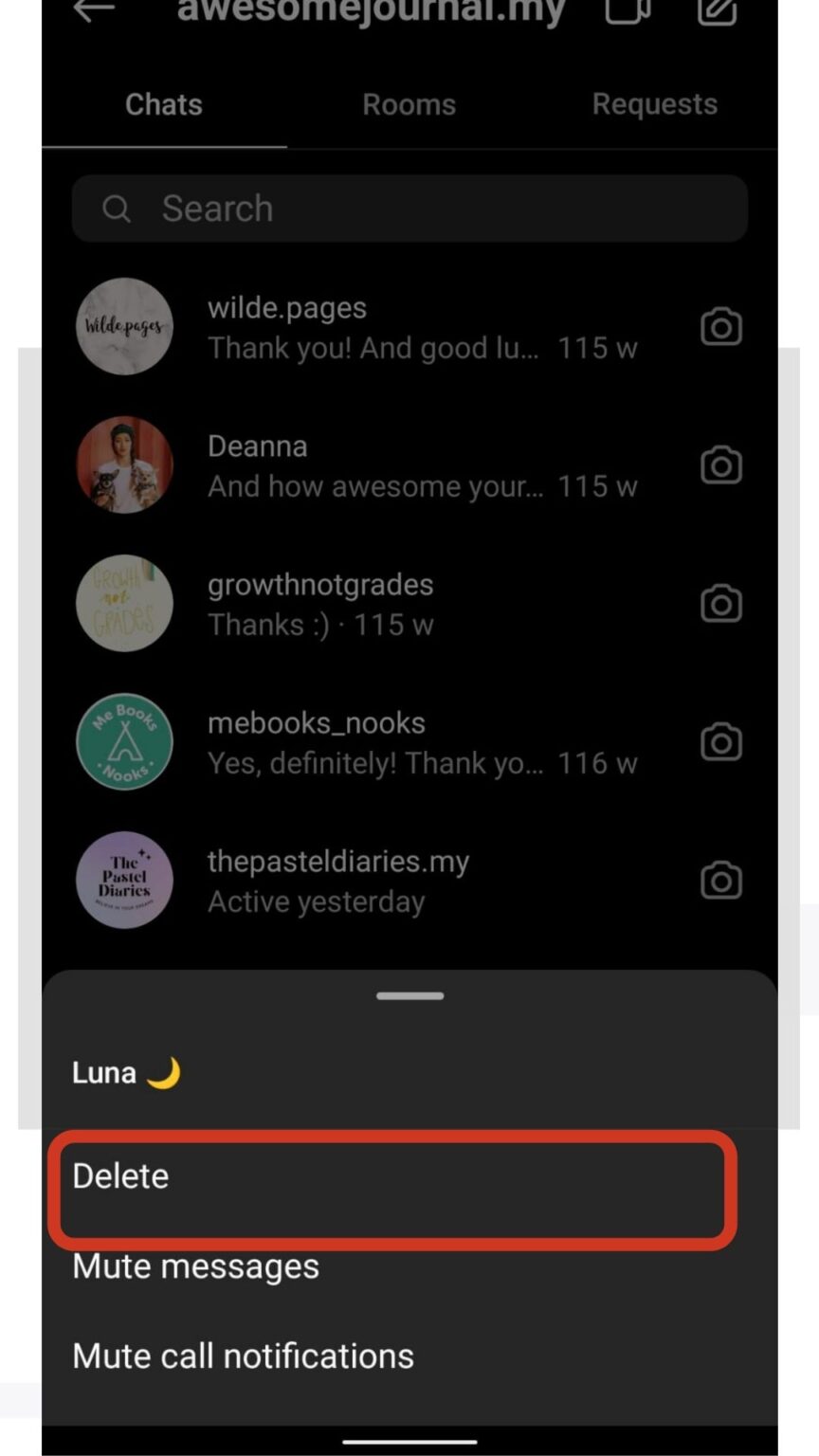A cleaned-up and detailed caption for the screenshot image:

---

This image is a cropped screenshot, apparently taken from a cell phone. It showcases a portion of a web page or app interface, as indicated by the incomplete URL "awesomejournal.my" visible at the top. The screenshot is cropped such that the back arrow is only partially visible.

The interface also includes an icon, which is partially cropped but seems to resemble a pencil, suggesting an editing feature. Below the URL, there are three tabs visible: "Chats," "Rooms," and "Requests." The "Chats" tab is highlighted and underlined, indicating the current selection in a bolder gray font against a black background, making it a bit challenging to read.

Further down, there's a search bar with a magnifying glass icon and the word "Search." Below this, a username "wildpages" (spelled W-I-L-D-E dot pages) is visible. A message below this handle reads: "thank you and good, L-U..." from 155 weeks ago. The Instagram logo, which looks like a camera, accompanies this message. 

Continuing, the name "Deanna" appears with the words "how awesome you are," possibly indicating a message or compliment in an inbox. 

Towards the bottom of the screenshot, various actions are listed including "Luna," accompanied by a crescent moon icon reminiscent of Sailor Moon. There is also a red rounded-edged square with the word "Delete," alongside options for "Mute Message" and "Call Notifications."

---